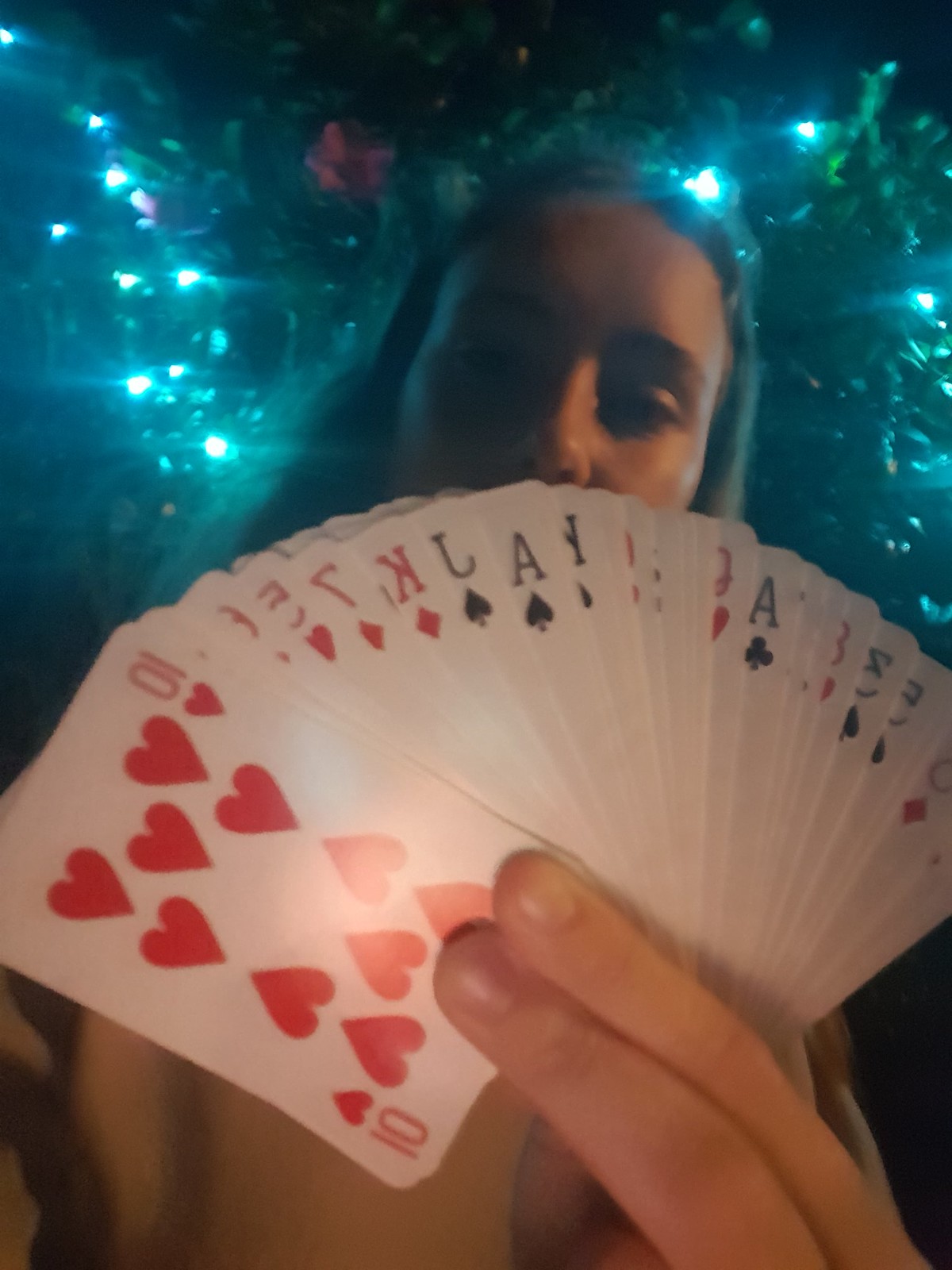A person is holding a large, fanned-out deck of cards in both hands, facing the camera. Their index and middle fingers are visible, grasping the cards firmly with their thumb at the back. The top card in the fan is the 10 of Hearts, distinctly marked with the number 10 in each corner and adorned with 10 red hearts. Among the visible cards, there is also a King of Diamonds, Jack of Spades, and an Ace of Spades, arranged without any specific pattern or sequence, suggesting a random assortment rather than a cohesive hand for a particular card game. The deck appears to contain over 20 cards.

The scene is set outdoors at night, but is well-lit, allowing clear visibility of the cards and surroundings. Behind the person, there are garden string lights that cast a bluish glow, illuminating a backdrop of lush tropical foliage, possibly hibiscus plants in bloom. The individual seems to be seated at a garden table, capturing a moment in a vibrant, night-time garden setting filled with summer flowers and decorative lighting. The image evokes a relaxed, outdoor evening atmosphere amidst a verdant garden.